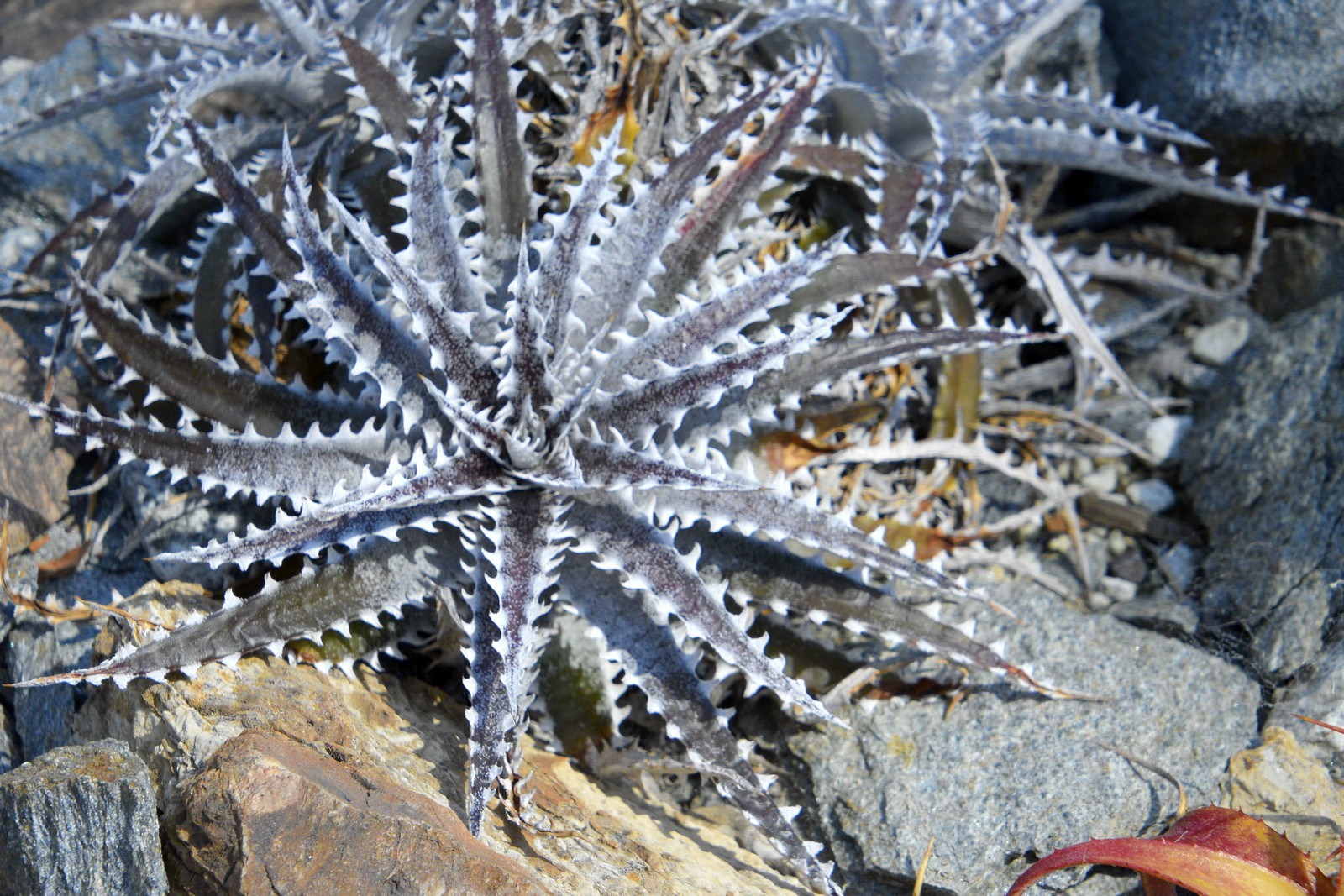In the center of the image, there is a striking plant with star-like symmetry, featuring long, spiky leaves that radiate outward in a concentric circle. The leaves are primarily white with jagged, tooth-like edges resembling shark's teeth, and their tips are tinged with dark green, almost black coloration. The plant is growing out of a cluster of varying rocks, including brown, gray, and black stones, creating a stark contrast with its sharp, pale foliage. Surrounding this prominent central plant are a few smaller ones of the same species, and scattered around the base are dried leaves, suggesting a dry, arid environment.